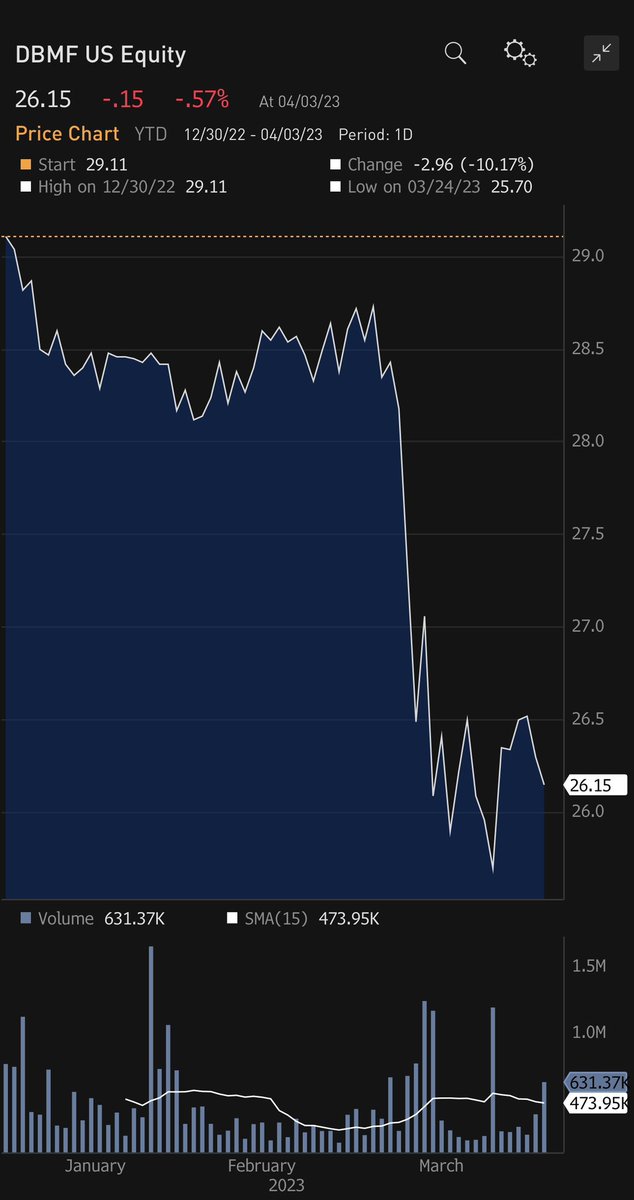A screenshot of a financial activity graph for DBMF U.S. Equity is displayed. At the top left, the current price is shown as $26.15. The price has decreased by $0.15, representing a 0.57% decline. The graph is labeled "Price Chart, YTD" (Year-To-Date). Various benchmark values are indicated on the graph: $12.30, $22.00, $2.40, $3.00, $23.00, with the starting point at $29.11. There has been a change of -$2.96, or a 10.17% decrease. Key notable points include the lowest value of $3.00, and the high values recorded on $12.30 and $22.00, with the peak at $29.11.